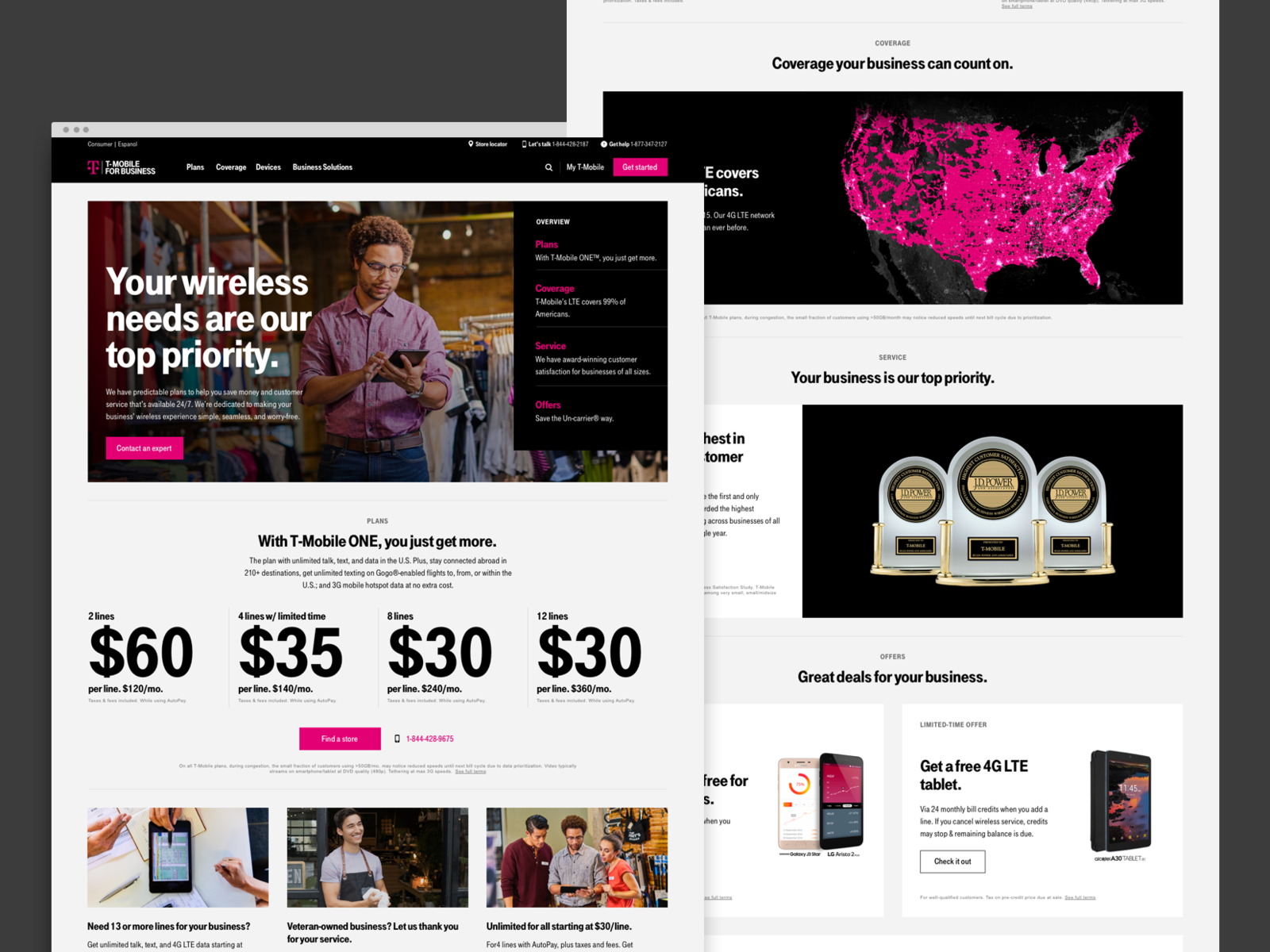A high-resolution promotional image features a man clad in a pink shirt, jeans, and glasses, standing against a minimalist white background for a clean, modern look. He holds an iPad displaying detailed information on various pricing plans: $60, $35, $30, and $30. In the background, a vibrant pink map is displayed with the text, "Coverage your business can count on, so your wireless needs are our top priority." 

On the iPad screen, a pink rectangle invites viewers to "Find More," and a phone number is prominently showcased. Accompanying this are three article headers: "Your Business Is Our Top Priority," "Great Deals for Your Business," and "Get a Free 4G LTE Tablet." Visual elements include two smartphones and a tablet, highlighting a "Limited Time Offer" for a free 4G LTE tablet. A white-gray rectangle at the bottom of the image features the call to action: "Check It Out."